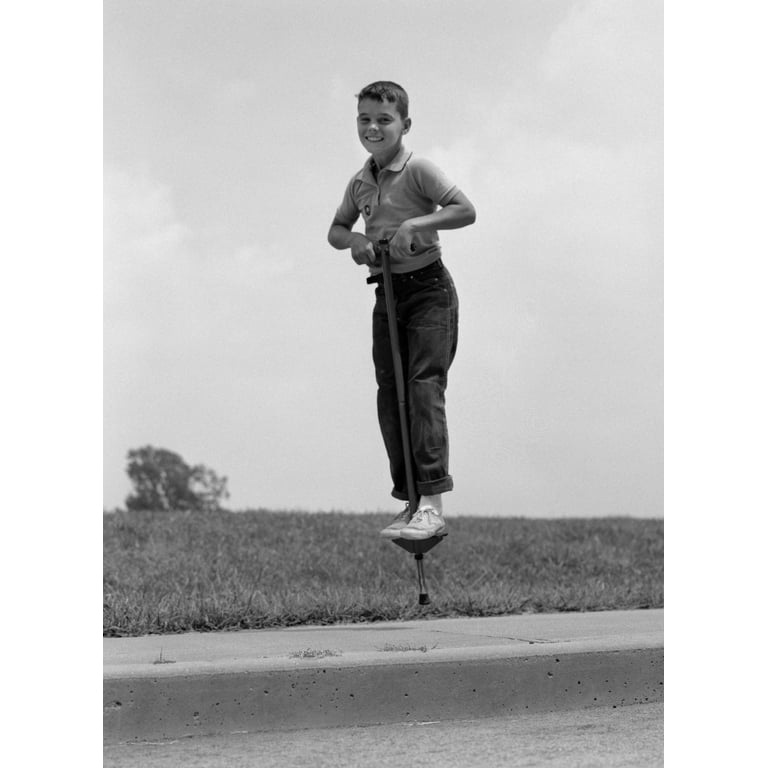This vintage image, likely from the 1950s or 60s, captures a young boy around 8 to 10 years old joyfully bouncing on a pogo stick. He has short brown hair and is dressed in a short-sleeved polo shirt tucked into brown pants or jeans, with white tennis shoes completing his outfit. The photo, vertically aligned and in black and white, freezes him mid-air with his hands gripping the handles of the pogo stick and his feet positioned on the footpegs. His bright smile reveals visible teeth as he looks directly at the camera, clearly enjoying himself. In the background, a solitary tree stands amidst an expansive grassy field, with a cloudy sky above adding to the nostalgic ambiance. The boy is playing along a sidewalk that's adjacent to a country road, emphasizing the idyllic and carefree moment captured in this timeless photograph.